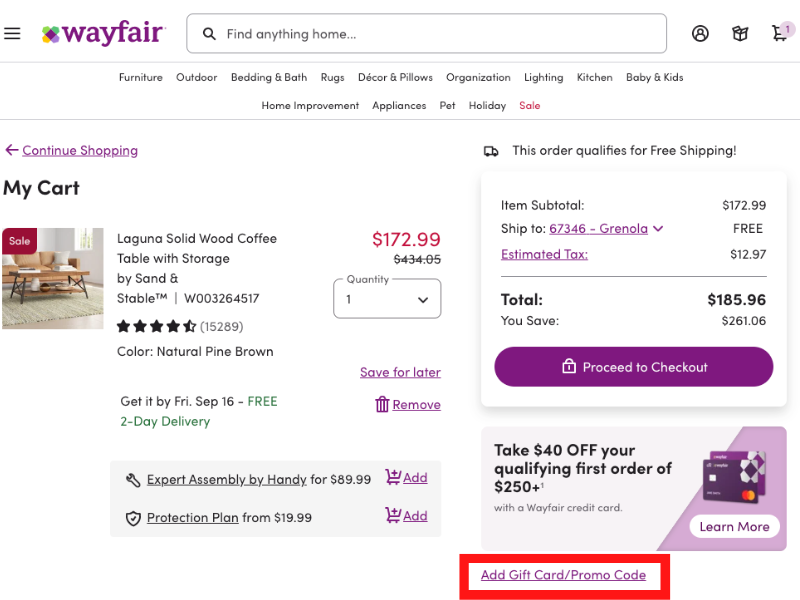**Detailed Caption:**

The image displays a webpage from the retail site Wayfair, known for its extensive catalog of home goods. In the top-left corner, the distinctive Wayfair logo is prominently featured in purple. Adjacent to the logo is a search bar with the placeholder text "Find Anything Home," inviting users to discover a wide array of home-related products.

Beneath the search bar, several category options are neatly listed to help users navigate the site: Furniture, Outdoor, Bedding & Bath, Rugs, Decor & Pillows, Organization, Lighting, Kitchen, Baby & Kids, Home Improvement, Appliances, Pet, Holiday, and Sale.

The content below these categories focuses on a specific product that a shopper is currently interested in. The "My Cart" section is displayed, highlighting the "Laguna Wood Coffee Table with Storage." A crisp image of the table is shown on the left side. To the right, the item's price is clearly marked at $172.99. Furthermore, the product boasts an impressive rating of four and a half stars and is described as having a natural pine brown color.

On the far right of the screen, the subtotal of the item is presented, accompanied by a prominent, clickable purple button labeled "Proceed to Checkout," encouraging the user to finalize their purchase.